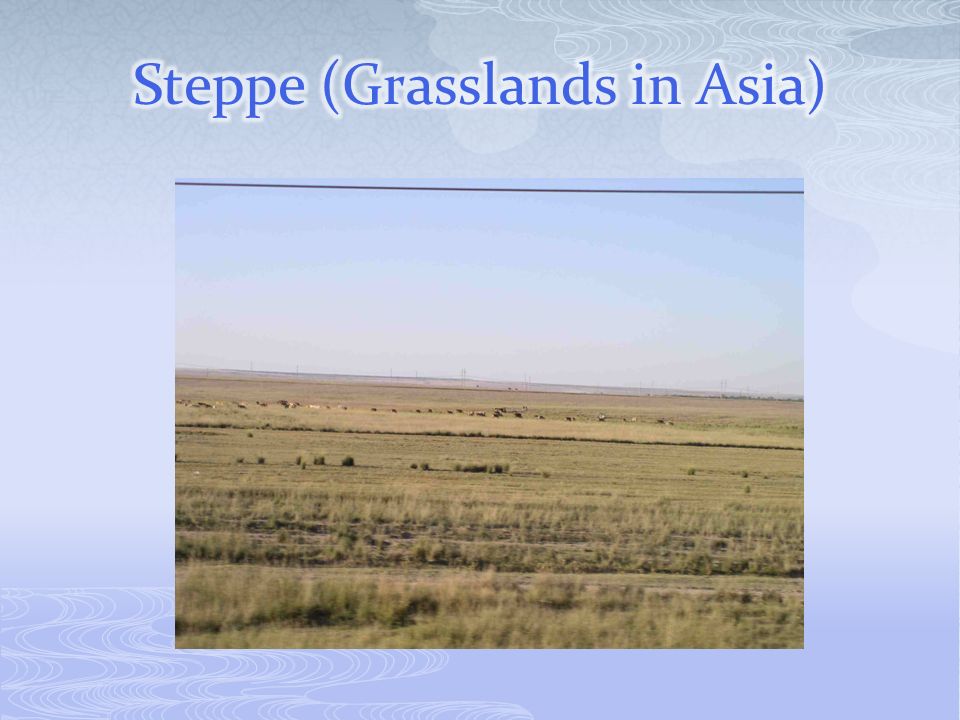This presentation slide, likely created in PowerPoint, showcases the steppes, also captioned as "grasslands in Asia." The title resides at the top of the slide, written in blue text with a white outline. The background features a gradient of blue that shifts from darker at the bottom to lighter at the top, adorned with wavy and swirl patterns in the upper right and lower left corners. Dominating the central portion is a large image of the steppes, vast plains characterized by short grasses predominantly in wheat hues with sparse patches of green. The flatlands extend to a clear, cloudless horizon. In the distant background, there might be animals, possibly cattle, and faintly visible cables, which could be power lines or components of a distant bridge. The overall color palette of the slide includes shades of blue, gray, white, lilac, and hints of green and black, lending a serene yet informative aesthetic to the presentation's depiction of Asian grasslands.